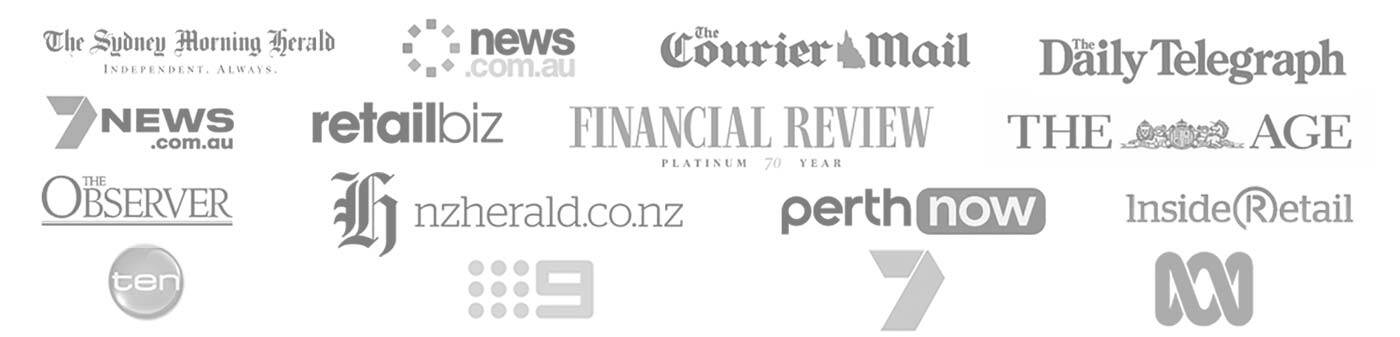This image depicts a grid of logos representing various media and news organizations, arranged in four rows. 

- **First Row (Left to Right):** 
  - The Sydney Morning Herald with the tagline "Independent. Always."
  - News.com.au
  - Courier Mail
  - Daily Telegraph

- **Second Row (Left to Right):**
  - 7news.com.au
  - Retail Biz
  - Financial Review Platinum (celebrating 70 years)
  - The Age, accompanied by an icon resembling a British crest

- **Third Row (Left to Right):**
  - The Observer
  - Another instance of The Age
  - NZ Herald (nzherald.co.nz)
  - Perth Now
  - Inside Retail

- **Fourth Row (Left to Right):**
  - Channel 10
  - A logo featuring six dots arranged in a cube shape
  - Channel 9
  - Channel 7
  - An icon combining uppercase 'M' and lowercase 'm' into one symbol